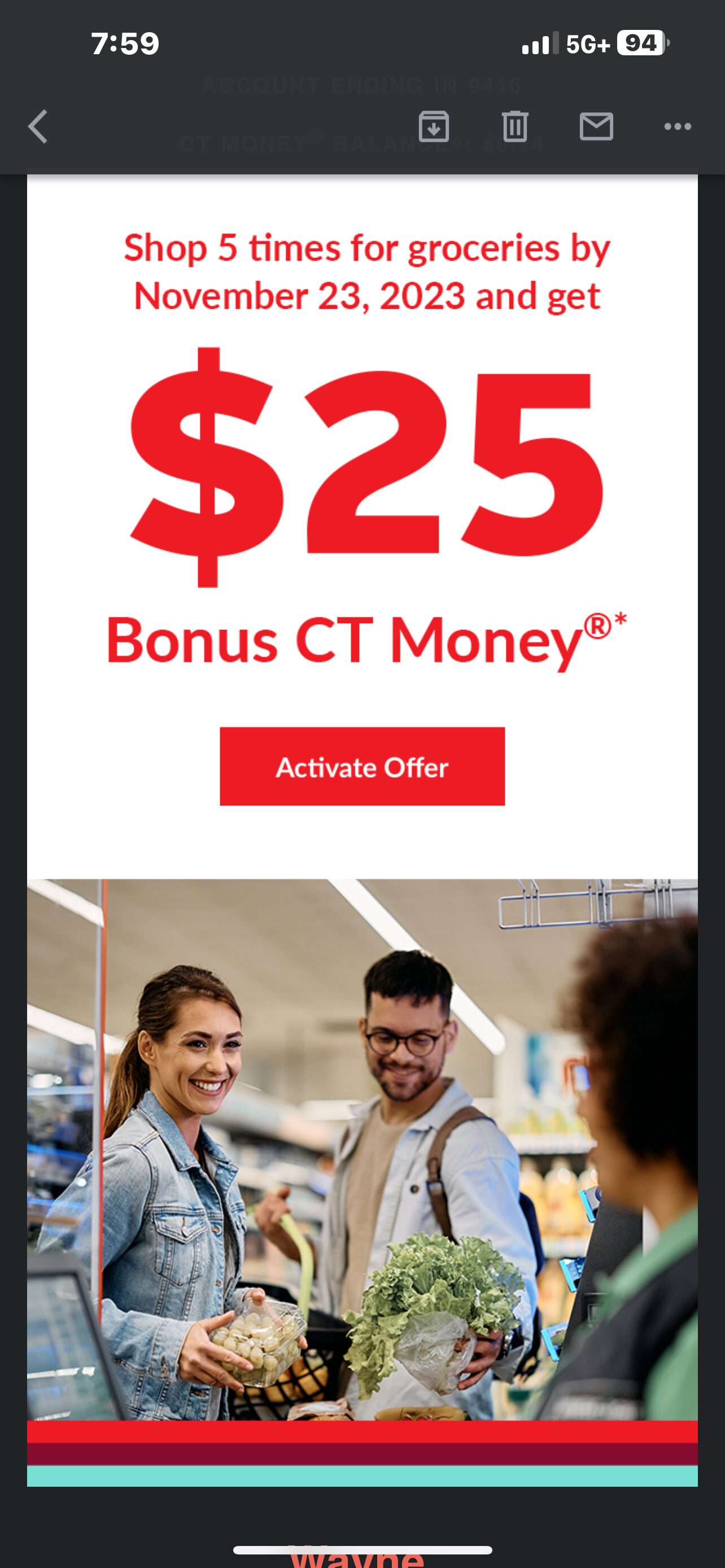A screenshot captured on a smartphone displays a large promotional pop-up within an unspecified app. The phone's status bar shows the time as 7:59, 4-5 bars for signal strength, 5G+ connectivity, and a battery at 94%. Below that, an interface bar includes a back button on the left, followed by icons for downloading, trash, email, and more options indicated by three dots.

Dominating the center of the screen is a prominent advertisement featuring a large white rectangle with bold red text announcing a promotional offer. The text reads: "Shop five times for groceries by November 23rd, 2023 and get $25 bonus CT Money" (with 'CT Money' marked as a registered trademark and an asterisk indicating further conditions). A striking red button below this text instructs users to 'Activate Offer,' written in white font.

Underneath the promotion, there's an image of a man and a woman at a grocery store checkout. The man, holding lettuce and wearing a backpack, has short hair, reading glasses, a scruffy beard, and a mustache. The woman beside him, sporting curly hair and glasses, a vest, and a green shirt, appears slightly blurry. To the right, another woman with a long ponytail is smiling widely and may be holding grapes in a plastic container.

At the bottom of the screen, several horizontal bars in orange, red, and a very light color span the width of the image. The word "Wayne" appears beneath these bars in orange text for an unclear reason.